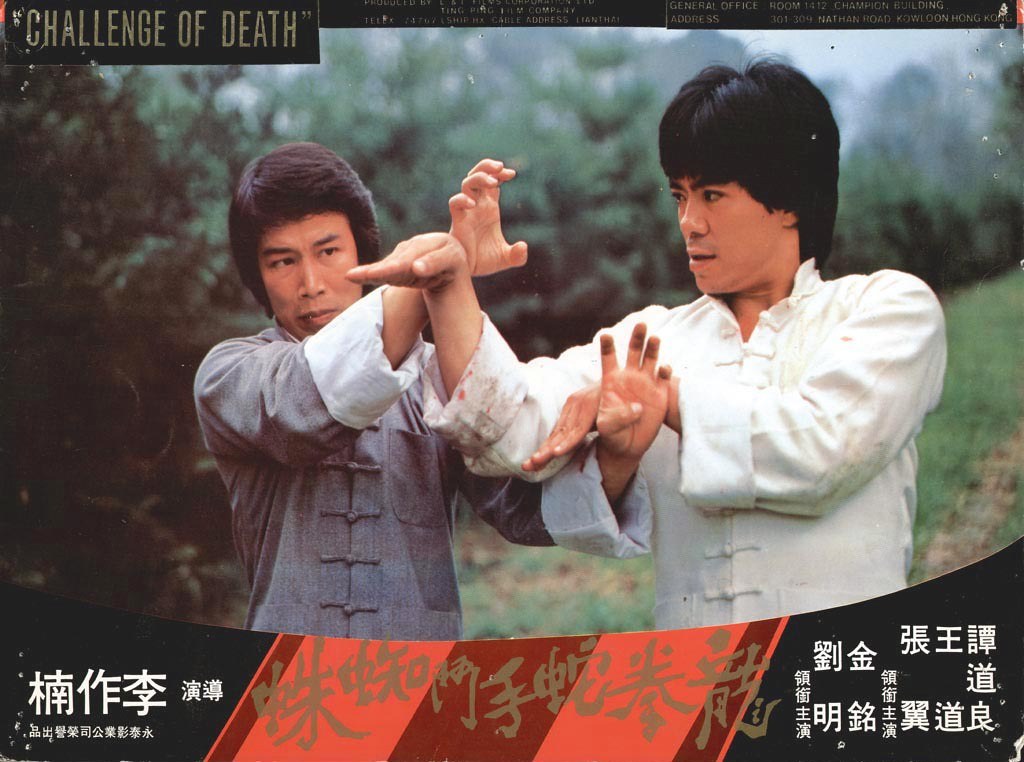The full-color image depicts two Asian gentlemen engaged in what appears to be a karate or kung fu martial arts bout. The scene unfolds outdoors in a natural setting amid grass and numerous trees, clearly during the daytime. The gentleman on the left is clad in a grayish top, while the one on the right sports a white top. At the upper left-hand corner of the image, the title "Challenge of Death" is prominently displayed in white text on a black background. Below this, Asian characters are featured against different backgrounds: white text against black in the corners, and gray text on a striped dark red and lighter red backdrop in the middle. This composition strongly suggests that the image could be a scene from a movie, likely a poster or promotional material for the film.